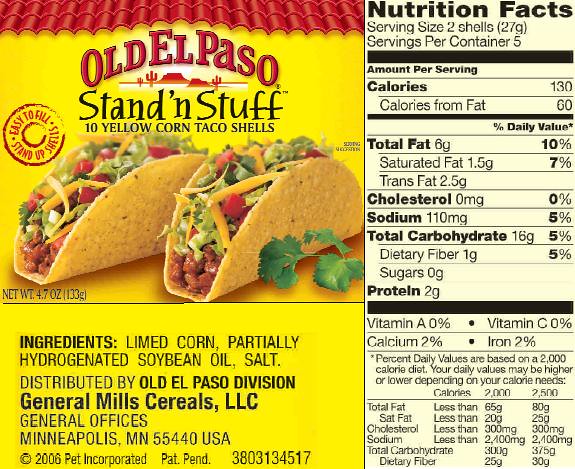This is a detailed description of a food label for Old El Paso Yellow Corn Taco Shells. The label is square-shaped, predominantly featuring a bright yellow background. Covering the top two-thirds of the label, there is Old El Paso’s distinctive curved red block print text set against the yellow, supplemented by a border resembling a red corrugated roof. A notable round logo declares, "Easy to Fill, Stand Up Shells." The illustration below this logo displays two taco shells, filled with what appears to be beef or beans, salad greens, tomatoes, and cheese.

The right third of the label, from top to bottom, is allocated to the nutrition facts, displayed in a pale yellow and black print. The serving size is listed as two shells, with five servings in the package, thus containing ten taco shells in total. Each serving accounts for 130 calories. 

Beneath the taco shells picture, separated by a thin black line, lies the ingredient list, which includes limed corn, partially hydrogenated soybean oil, and salt. The label also mentions that the product is distributed by the Old El Paso Division of General Mills Cereals, LLC, with general offices based in Minneapolis, Minnesota.